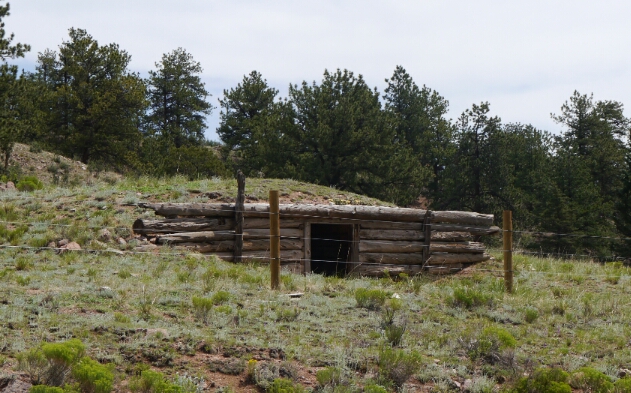The photo depicts a rustic, underground log cabin or bunker carved into a grassy hillside. The structure is primarily made of wood, with logs lining the entrance and forming the walls. The doorway is a dark, black opening that beckons with mystery, offering no hint of what lies within. The surrounding grassy area is uneven and appears unmaintained, featuring various types of grass, some reaching up to six inches in height and darker in color. In front of the entryway, a wire fence with several wooden posts stands, possibly supported by barbed wire. The roof of the cabin is composed of logs covered with a dome-shaped mound of dirt, in which grass has sprouted, blending the structure seamlessly into its environment.

The scene is set at the peak of the hill, under a cloudy daytime sky. Mature pine trees encircle the area, adding to the secluded and natural feel. There's also mention of a small square lookout window incorporated into the cabin's design. The overall color palette is dominated by shades of green and brown, with some hints of yellow, creating a harmonious balance between the man-made and natural elements. No people are visible in this solitary and serene setting.